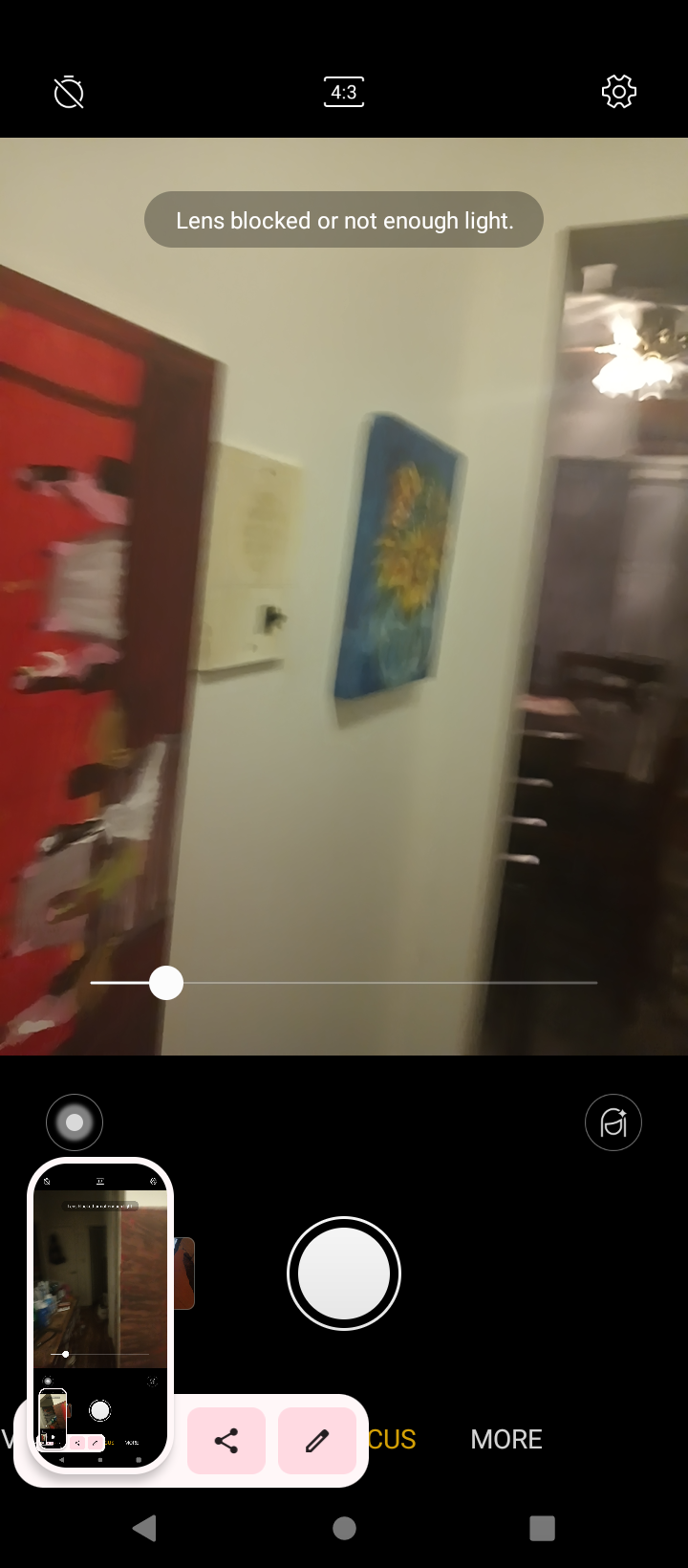This image is a blurry screenshot of a phone's camera interface, captured during a paused video recording. At the top of the screen, a notice reads "Lens blocked or not enough light," indicating poor visibility. The interface shows a control line with a white dot towards the left, suggesting the video is paused. The visible scene seems to be the entrance hallway of an apartment with a white wall. On this wall, there is a small intercom speaker next to a rectangular painting, which appears abstract and might depict people sitting at tables. Further to the right of the speaker, a framed image of yellow flowers in a clear vase is visible against a blue background. In the distance, a glimpse into another room shows a dining chair and a blurry white light from a fan on the ceiling.